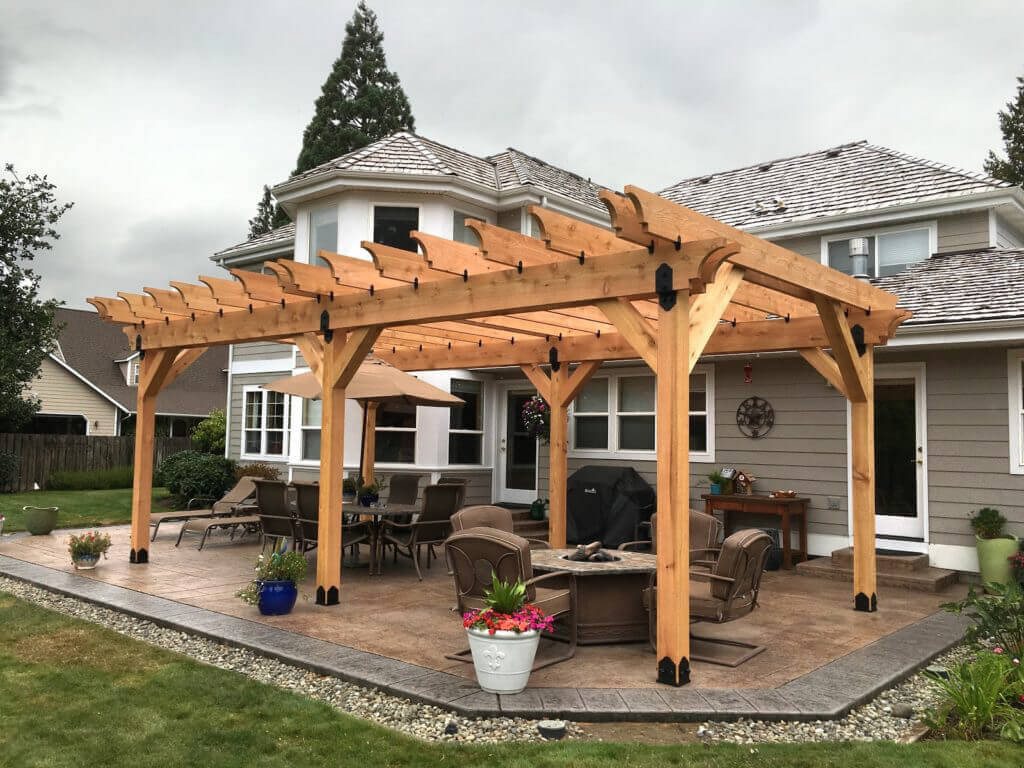This image captures the backyard scene of a modern, two-story house painted in gray with horizontal siding and white trim around multiple windows. The house's roof and walls sport a sleek gray tone, adding a contemporary vibe. A notable feature in the backyard is a brand new, wooden pergola without a cover, designed to potentially support future flowering plants or provide shaded seating. Underneath the pergola is a cozy seating area with cushioned chairs around a table, as well as additional lawn chairs spread across the patio. There is also a distinct, tiled patio area bordered by small decorative rocks and adorned with various potted plants and flowers. Adjacent to the house wall sits a covered barbecue grill next to a small side table with a decorative element on it. Further to the right, four chairs encircle a fire pit, offering a perfect spot for gatherings. The well-maintained lawn is flanked by various bushes, flowers, and trees, with another neighboring house visible to the left behind a wooden picket fence. The sky above is overcast, hinting at potential rainfall, enhancing the tranquil atmosphere of this picturesque backyard.